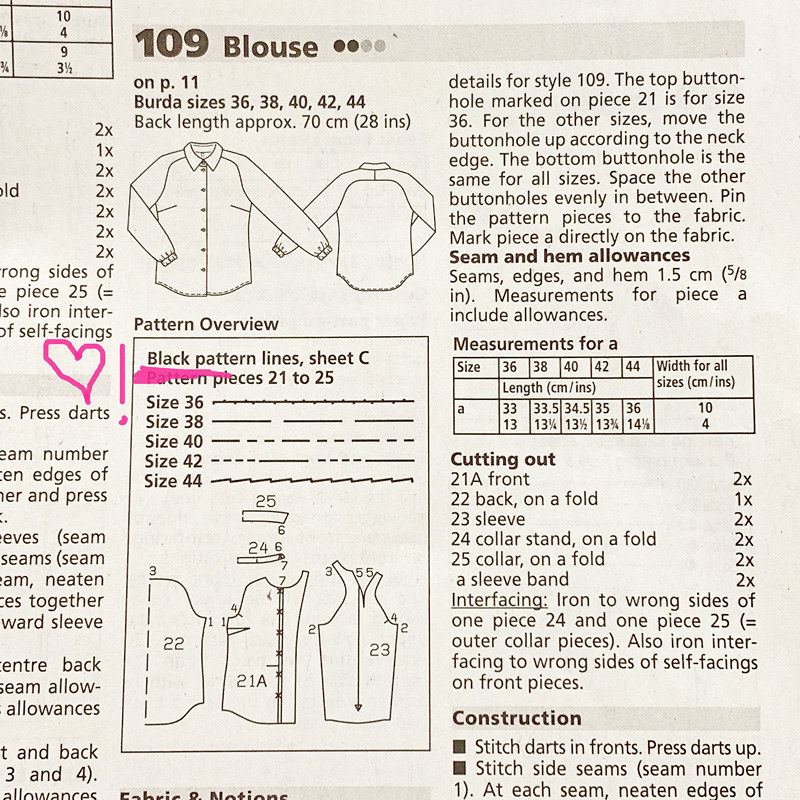The image is a detailed snippet from a sewing pattern book, featuring instructions for creating a blouse labeled as "109 Blouse." The piece is a horizontally rectangular, off-white page highlighted with pink marks. It provides comprehensive information on constructing a blouse available in Burda sizes 36, 38, 40, 42, and 44, with a back length of approximately 28 inches (70 centimeters). 

The top section of the image displays the blouse design through illustrations of both the front and back views of the garment, showcasing structured lines around the chest area, pleated cuffs, and unique design features for the shoulders and back. A detailed pattern overview is included, illustrating the various pieces required to assemble the blouse. Someone has used a pink highlighter to underline the phrase "black pattern" and has drawn a pink heart with an exclamation point next to it, indicating the importance of this detail. 

The right side of the page offers extensive details on the measurements, sizes, and instructions for cutting and stitching the blouse, although it does not provide the complete set of instructions in the photograph. The nature of the page, with its segmented details and illustrations, suggests it comes from a specialized pattern book used by seamstresses and designers to create custom clothing.